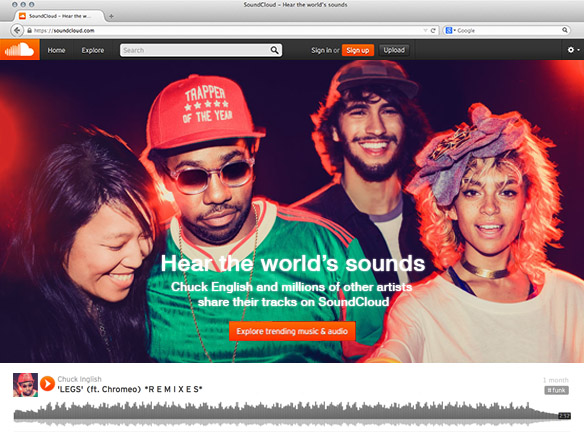The image is a screenshot of a website displayed on a computer screen. The top section of the screen is gray. Below this, the browser tab is open, showing the website's title and the URL in a search box. To the right of the URL, there is another search box. 

On the main part of the page is an image featuring four people. On the left side is an Asian woman with black hair, who is smiling and looking down towards the center of the image. To her right is an African man wearing a red ball cap, a green shirt with red stripes down the shoulders, and sunglasses. He has a short dark beard and mustache. Further to the right is a white man with a shoulder-length hairstyle, a black mustache and beard, and a purple hat. He is dressed in a white jacket over a black jacket and a white shirt. 

On the far right is a woman with shoulder-length, fiery orange and red hair, wearing a golden necklace and a white shirt. The background of the image is predominantly black, with some red accents on the left and right edges.